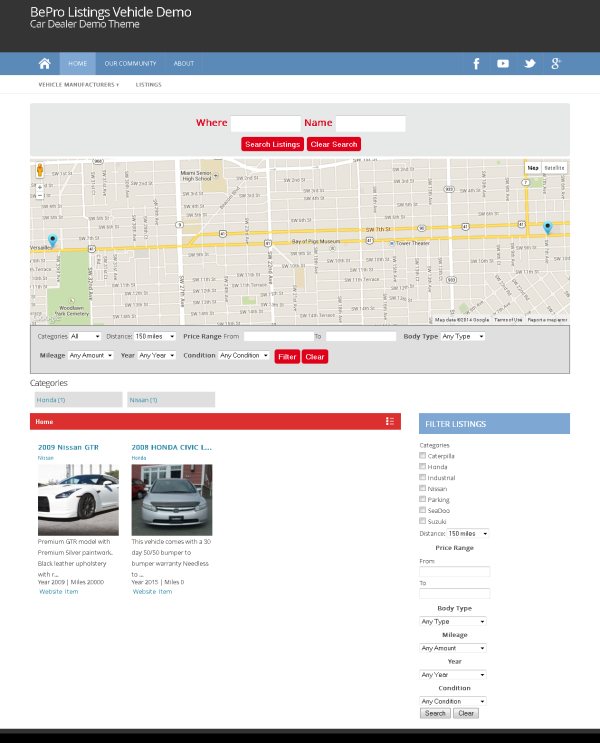The image showcases an interface for the Bepro Listings Vehicle Demo, a platform designed to help users locate car dealers offering promotional demonstrations of specific vehicles. At the center of the screen, a zoomable map displays dealership locations, enabling users to adjust their view to focus on particular areas. Above the map, a dropdown menu allows users to filter results by vehicle manufacturers, while next to it, a search bar accommodates specific words and names for refined queries.

On the bottom right of the screen, a comprehensive search module offers additional filtering options, such as brand preferences, parking facilities, price ranges, body types, mileage, and the year of the vehicle. To the left of this module, thumbnail images of two vehicles—a Nissan GTR and a Honda Civic—are shown with brief overviews and clickable links for more detailed information.

Overall, the Bepro Listings Vehicle Demo provides a streamlined and user-friendly interface for car enthusiasts to discover and arrange test drives with ease.